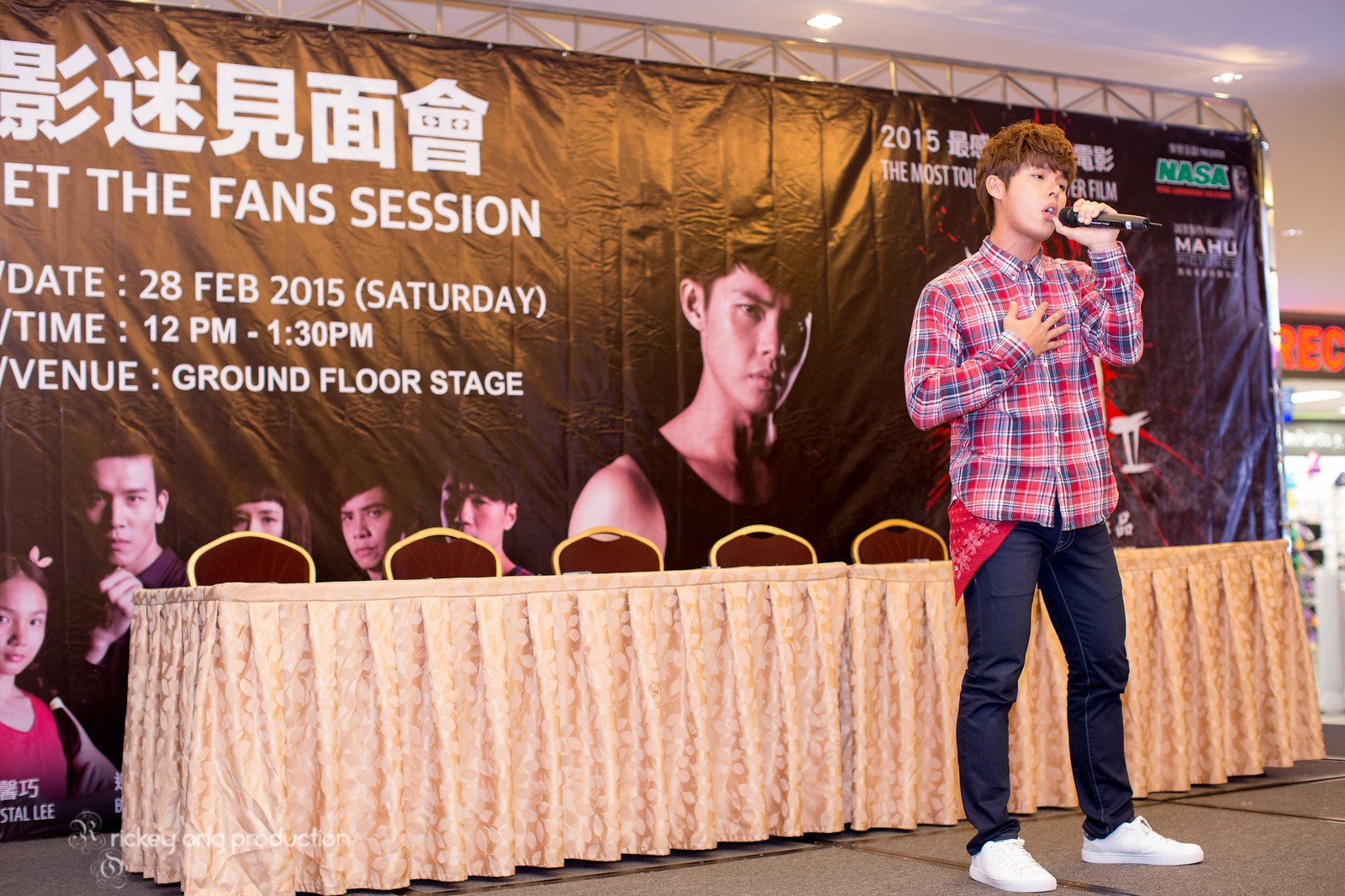This indoor photograph captures a young Asian man, likely in his late teens or early 20s, enthusiastically singing into a microphone while standing on a platform. He sports a medium shaggy haircut and is dressed in a red, blue, and white plaid shirt, with a red handkerchief tucked into his right pocket. His outfit is completed with blue jeans and white sneakers. In his left hand, he holds the microphone up to his mouth, while his right hand rests near his chest. 

Behind him, there is a large black banner with both Asian and English text, advertising a "Meet the Fan Session" scheduled for February 28, 2015, from 12 p.m. to 1:30 p.m. The banner also features images of Asian individuals, including one in the center and a group of others alongside. A skirted table with about five visible chairs stands in the background, adding context to the event's setting on the ground floor stage.